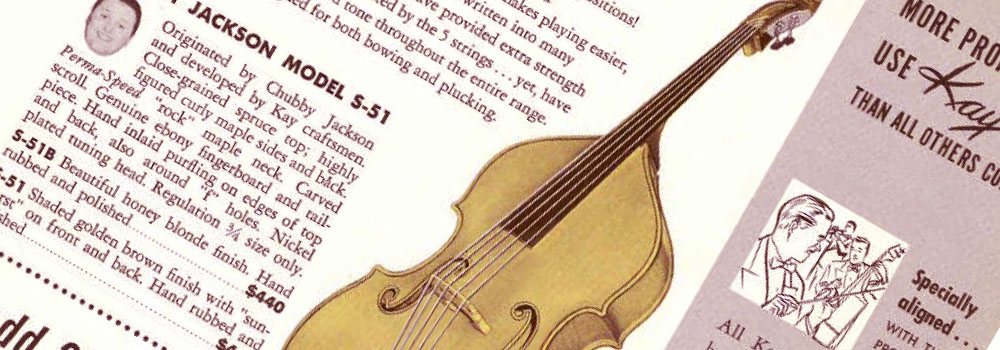This image displays a scanned portion of an old musical instrument catalog. The page prominently features a detailed drawing of a violin-type instrument against a dual-toned background, with white on the left and a brownish-pink hue to the right. The visible text to the left promotes the "Jackson Model S-51," developed by Chubby Jackson and Kay Craftsman. It boasts a close-grain spruce top, highly figured curly maple sides and back, a perma-speed rock maple neck, a carved scroll, and a genuine ebony fingerboard and tailpiece. Additional features include hand-inlaid purfling on the edges of the top-plated tuning head, with the instrument available in a regulation 3/4 size only. Particularly highlighted is the "S-51B" model, which is described as having a beautiful honey blonde finish, hand rubbed and polished, all priced at $440.